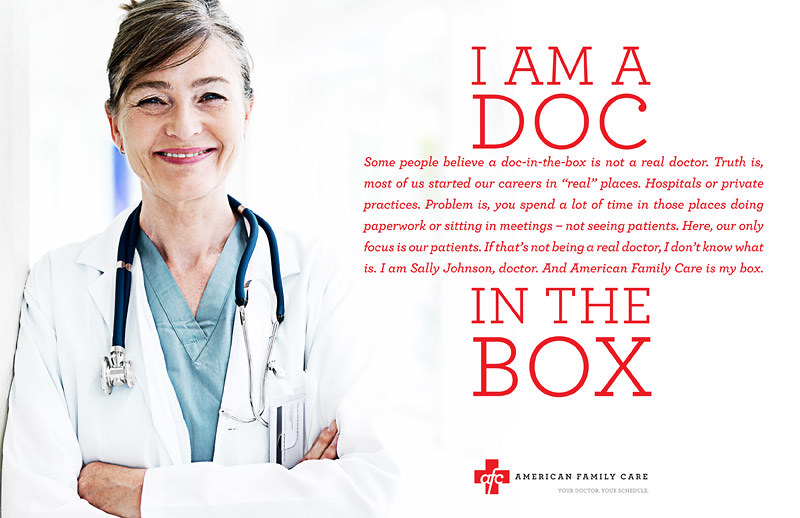The advertisement for American Family Care features an older, smiling female doctor standing proudly to the left of the image. She appears to be in her early 60s, with grayish-brown hair tied up in a bun, and is wearing a white lab coat over a green scrub shirt, with a stethoscope draped around her neck. Her arms are folded confidently across her chest. Beside her, in bold red letters against a clean, white background, it reads "I am a doc." A lengthy paragraph below elaborates on the misconceptions about "docs in a box," emphasizing that many of these doctors began their careers in traditional medical settings, like hospitals or private practices, but shifted to focus more directly on patient care without administrative distractions. The text expresses pride in this focused approach, concluding with the doctor's name, Sally Johnson, and a declaration that "American Family Care is my box." At the bottom of the image, the tagline "American Family Care" is prominently displayed, along with their slogan "Your doctor, your schedule," adjacent to their red cross logo marked with the letters AFC.